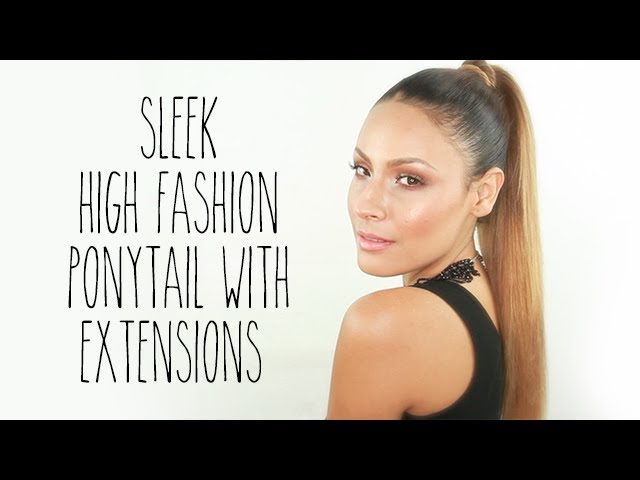This image, reminiscent of an advertisement, features a young woman, possibly in her 20s or 30s, with slightly darker, olive-toned skin. She is gazing over her shoulder at the camera, her long brown hair neatly styled into a high ponytail adorned with blondish accents. Her hair is sleek and accentuated with extensions, giving it a high-fashion appeal. She has light makeup, small brown eyes with long lashes, perfectly arched eyebrows, and wears pink lip gloss on her thin lips. Clad in a black tank top and a black necklace, her appearance is polished and stylish. Against a white background bordered by black bars on the top and bottom, a handwritten style font on the left reads, "Sleek High Fashion Ponytail with Extensions." This high-quality, professional image likely serves as an advertisement for hair extensions or could be used in a hair salon as an example of a trendy hairstyle.